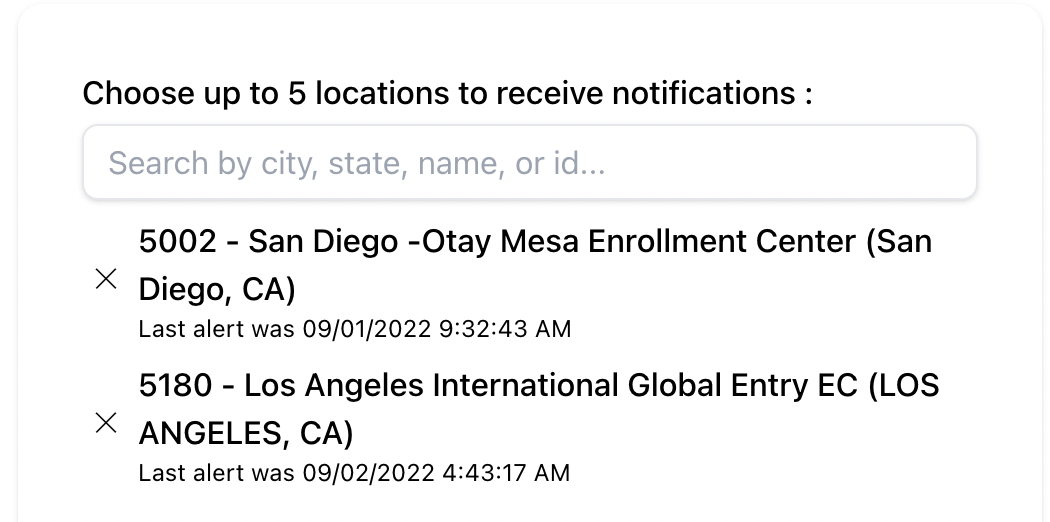The image is a horizontally oriented rectangle with a thin gray border along its left, top, and right edges, but no border at the bottom. The background within this bordered area is white. 

At the top of the image, there is a black text caption that reads, "Choose up to five locations to receive notifications." Below this, a gray outlined rectangular box contains a search field labeled "Search by city, state, name, or ID."

Underneath the search box, the first entry appears: 
"5002-San Diego-Otay Mesa Enrollment Center, San Diego, California," followed by an 'X' icon to the left of it. At the bottom of this entry, it notes: "Last alert was 09/01/2022 at 9:32:43 AM."

Further down, there is a second entry:
"5180 Los Angeles International Global Entry EC, Los Angeles, California," also with an 'X' icon to its left. The note at the bottom of this entry states: "Last alert was 09/02/2022 at 4:43:17 AM."

There are no other notable elements within the image.